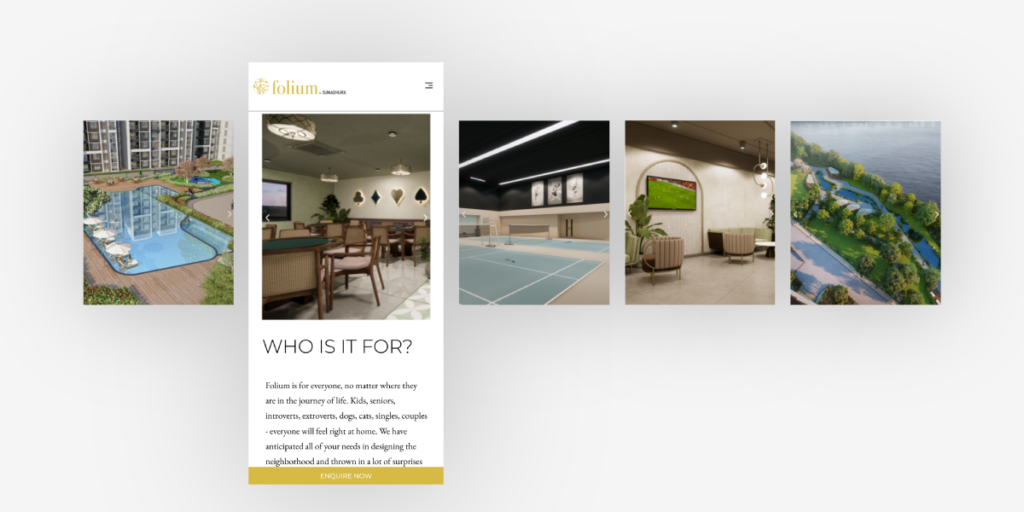The image features a light gray background with five small, horizontally aligned tiles in the center. Each tile represents a different aspect of a residential building, potentially an apartment complex. The first tile showcases a community pool, suggesting a recreational area for residents. The second tile, labeled "Folium," includes text that reads "Who is it for," and depicts a community sitting area designed for social gatherings. The third tile highlights an indoor tennis court, providing insight into the building's recreational facilities. The fourth tile showcases another community sitting area, resembling a lobby, which implies a welcoming entrance or common space. The final tile presents the landscape outside the building, featuring a body of water, a walkway, and abundant greenery with shrubs and trees. These images are designed to be interactive, allowing users to click or hover for more detailed information about each feature.